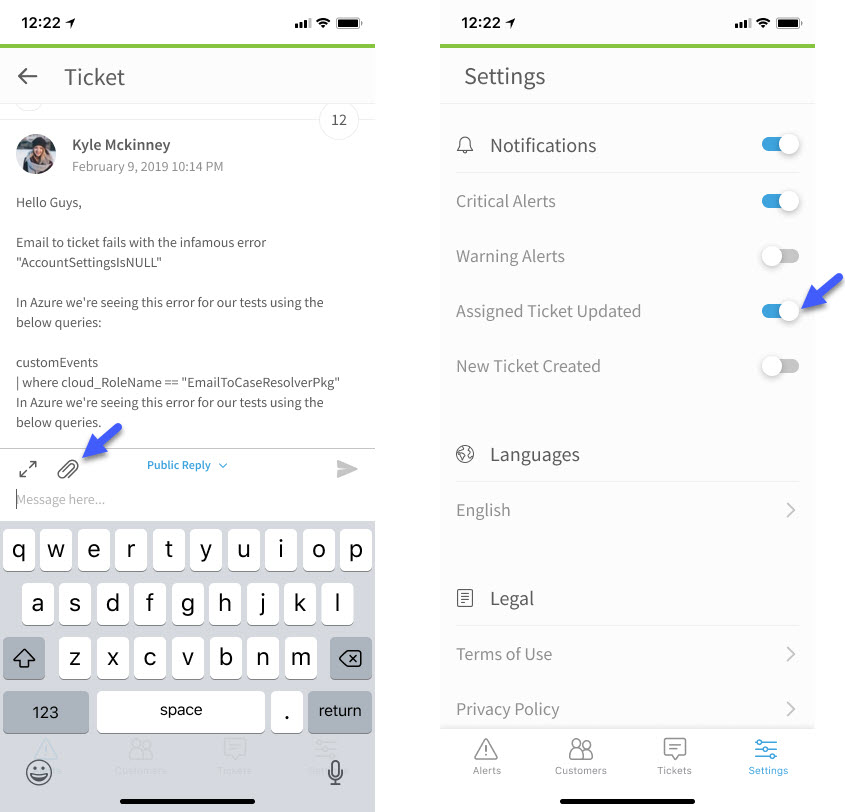The image features two different screenshots:

**Left Screenshot:**

- The top status bar shows the time "12:22" in bold black text, along with cellular signal strength (three out of four bars), a Wi-Fi symbol, and a battery icon.
- There is a dark green banner with a small bezel, featuring a dark black back arrow pointing to the left and the word "Ticket" in gray.
- Below the banner is a profile picture of a woman with shoulder-length blonde hair, wearing a black toboggan and a gray and black coat.
- Next to the profile picture, there's a white circle with the number "12" inside. The person's name, "Kyle McKinney," is written in bold black text, while "February 9th 2019, 10:14 p.m." is in gray text beneath it.
- The message reads: "Hello, hello guys, email to ticket fails with the infamous error 'account settings is null.'" The message continues on a new line: "In Azure, we are seeing this error for our tests using the below queries." Following this is: "Custom events where cloud_role_name == 'email_to_case_revolver_PKG'." 
- Below the text, there are two black error icons slanted to the side, accompanied by a slanted paper clip.

**Right Screenshot:**

- The top portion displays a settings page with notifications and alert options:
  - A dark blue arrow points to 'Assigned ticket updated,' which is turned on.
  - Notifications icons, including a bell, show that 'Critical alerts' are turned on while 'Warning alerts' are turned off.
  - 'New ticket created' is turned off.
  - 'Language' is displayed in black text, with "English" in gray beneath it.
  - Under 'Legal,' there are options for 'Terms of use' and 'Privacy policy,' each with a right-facing arrow next to them. There is also an arrow pointing right next to 'English.'
- The bottom of the screenshot features a text message field with a cursor inside and the QWERTY keyboard from a tablet or smartphone displayed.
- There is an arrow pointing to the right next to a gray icon and a dark blue arrow pointing towards a centered paper clip. Additionally, there is a hyperlinked text in blue with a down arrow.